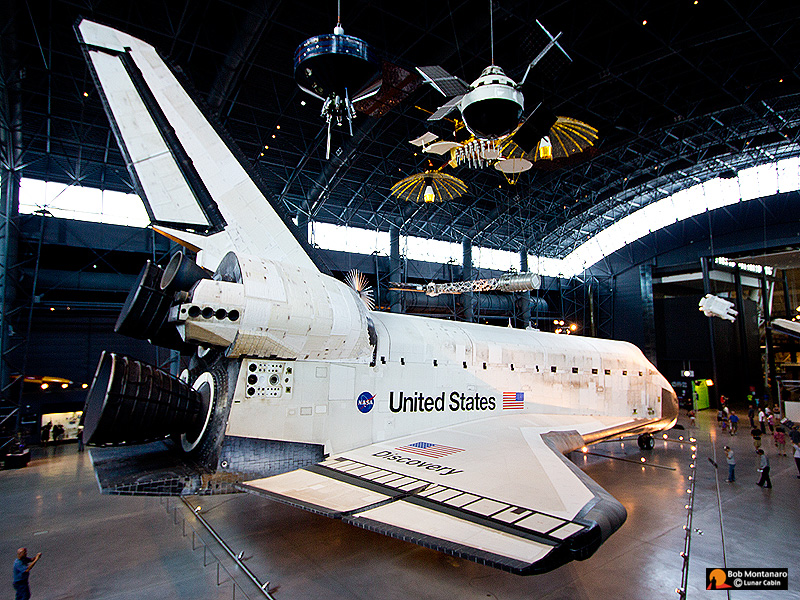Caption:

Inside the humongous hangar of the Smithsonian's Air and Space Museum in Washington, D.C., the Space Shuttle Discovery stands proudly on display. This impressive white spacecraft, reminiscent of an airplane with its tail fin and side wings, shows signs of wear on its exterior. "United States" is emblazoned on its side in black lettering, accompanied by the American flag to the right and the NASA logo to the left. The tail fin also features the American flag above the name "Discovery." The shuttle is equipped with three or four black rocket boosters on its back. The exhibit space is framed by a silver metal fence with some gold tones, and an arched roof with a dark ceiling and windows along the top edges of the walls. People are walking around the cordoned-off area, marveling at the historic spacecraft. Suspended overhead, a few satellites add to the allure of this vast, museum-like hangar.